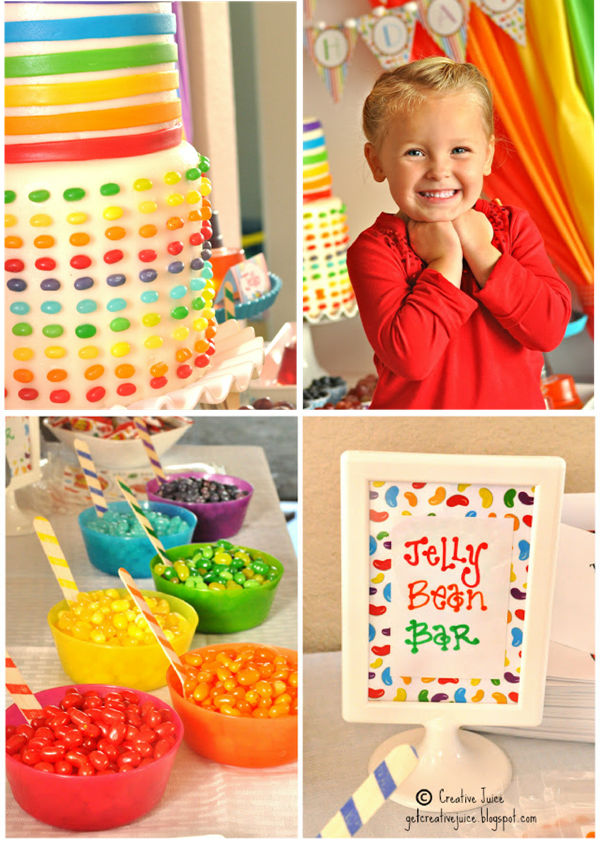The image is a vibrant collage of four different photographs showcasing a colorful, jelly bean-themed birthday celebration. The top left photo features a close-up of a white frosted birthday cake adorned with vertical rainbow stripes on the upper tier and a cascade of rainbow-colored jelly beans on the bottom tier. To the right, the top right photo captures a cheerful Caucasian child with blonde hair and a wide smile, wearing a red shirt and standing in front of the cake. Behind the child, there's a festive "Happy Birthday" banner and a curtain with rainbow colors. The bottom left image displays six bowls, each in a different color of the rainbow, filled with matching jelly beans—red in red, orange in orange, yellow in yellow, green in green, blue in blue, and purple in purple—arranged neatly on a table. The bottom right photo shows a framed sign that reads "Jelly Bean Bar" on a white ceramic stand. In the lower corner of the overall image, there is a copyright notice for "Creative Juice" and a reference to the blog getcreativejuice.blogspot.com. This lively composition captures the essence of a joyful, rainbow-themed birthday party.